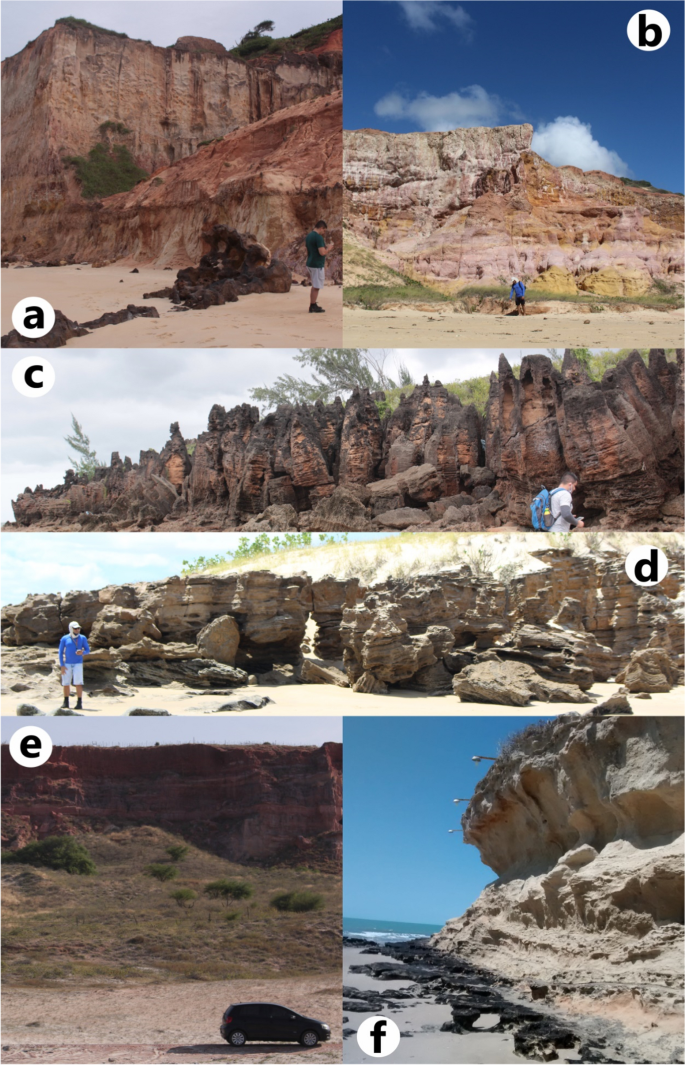This is a collage of six color photographs taken outside during the day, labeled A through F, each depicting various desert scenes dominated by rock formations:

- **Photo A** showcases a large rock formation in the desert with a person in a green shirt and gray shorts standing in the right corner, viewed from the side, looking away.
- **Photo B** features a very large rock formation under a blue sky with white clouds. There is a person wearing a blue shirt, standing far away in the center.
- **Photo C** presents a long, craggy rock formation. At the bottom of this photo, a person with a blue backpack, white shirt with gray sleeves, is facing right from the side.
- **Photo D** depicts another long rock formation with a person in the left corner. This person is outfitted in a blue shirt, blue jean shorts, and a white hat, facing right.
- **Photo E** shows a large mountain rock formation with greenery in the foreground and a gravel road with a black SUV parked to the right.
- **Photo F** is a sandy rock formation at a beach, featuring three lights hanging over the top, oriented to the left.

These images collectively emphasize the grandeur and variety of rocky desert landscapes, highlighting the presence of individuals exploring these terrains.